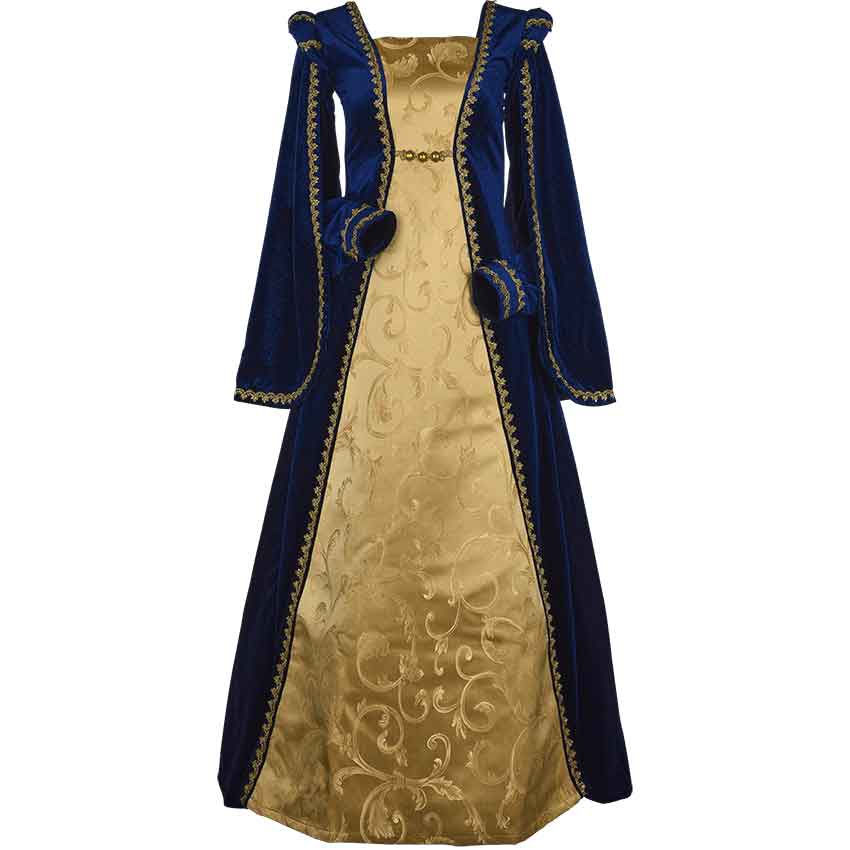The image depicts a highly ornate medieval-style dress, evocative of nobility, possibly worn by a queen or someone of high rank. The dress itself is a rich gold color, featuring intricate curly cue stitchings that extend from the neckline down to the hem, forming a silhouette reminiscent of a decanter. Wrapped around the shoulders, the ensemble includes a deeply dark royal navy blue garment, likely made of velvet or felt, adorned with elaborate brocade along the cape and arm sleeves. The sleeves are winged and capped off with gold embroidery at the cuffs. The overall craftsmanship conveys a high level of opulence and sophistication, hinting at its potential use in a theater production or its display in a museum.